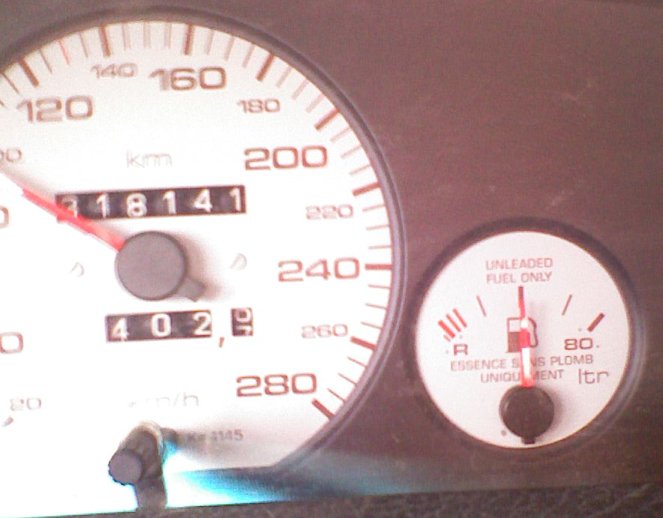The image features an extreme close-up of a vehicle’s dashboard. Prominently displayed on the left is a white-background, circular speedometer, partially cut off on its left side, showing speeds listed in kilometers per hour. The dial is pointed near 100 km/h, with the next visible number being 120. The speedometer's range extends up to 280 km/h. Below the speedometer, the vehicle's mileage reads 318141, with an additional smaller odometer showing 402. On the right side of the image, a fuel gauge reads, "Unleaded Fuel Only," highlighted by a red needle positioned centrally. The dashboard, bathed in black, gray, and red colors, suggests the photo was taken inside a car during the day.